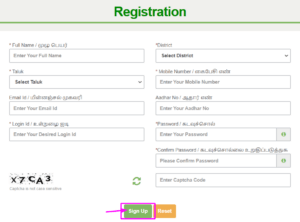The image is slightly wider than it is tall, approximately by 30%. It appears to be a screenshot or a mockup of a registration section from either a website or an application. 

At the top of the image, there is a gray background that occupies about 20% of the image. Just beneath this, a horizontal green line extends across the width, and centrally placed above this line in dark green text is the word "Registration".

On the left-hand side, several input fields are listed vertically. The first field is labeled "Full Name" with a required field indicator denoted by a star. Below this is an input box with placeholder text reading "Enter your full name". There are three more similar input fields beneath this, each with their own labels, although these specific labels are not clearly readable.

The right-hand side contains six additional input boxes arranged vertically. At the bottom left of the left-hand column, there is a CAPTCHA field displaying the code "X7CA3", which users must enter to verify they are human.

Centered at the bottom of the image is a green button with white text that says "Sign Up". To its right is an orange button with white text labeled "Reset".

A fuchsia-colored overlay highlights the "Sign Up" button, with a drawn arrow pointing towards it from the left side, likely to emphasize the button’s importance or guide user action.